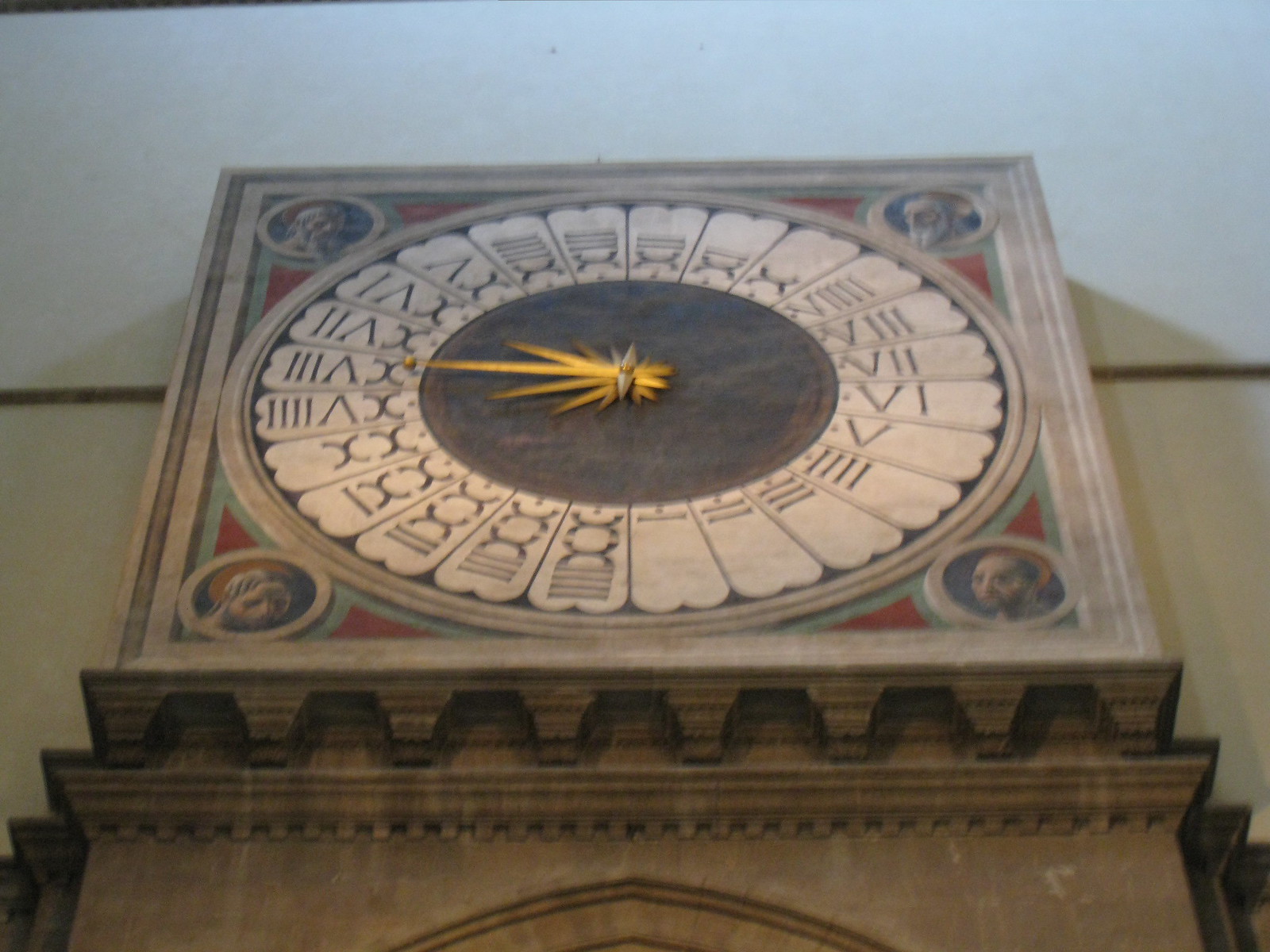The image showcases the top portion of a grandfather clock, captured from an upward angle that reveals both the underside and the front of the clock against a background featuring a painted white wall and a matching white ceiling. There is brownish or gold-colored edging between the wall and ceiling that frames the clock. The base of the clock is crafted from stylized wood with a decorative edging and a mantelpiece that progressively widens towards the bottom, where intricate designs are just beginning to emerge.

The clock face, which appears ancient or historical, is adorned with Roman numerals arranged unusually—starting at 1 and moving counterclockwise, extending potentially up to 25, resembling a sundial. The clock’s centerpiece is black with rich golden artwork, featuring intricate figures at each corner, framed in reddish and greenish hues that form a square around the round clock face. Golden clock hands, resembling sun rays, add to the ornamental allure of this distinctive timepiece.